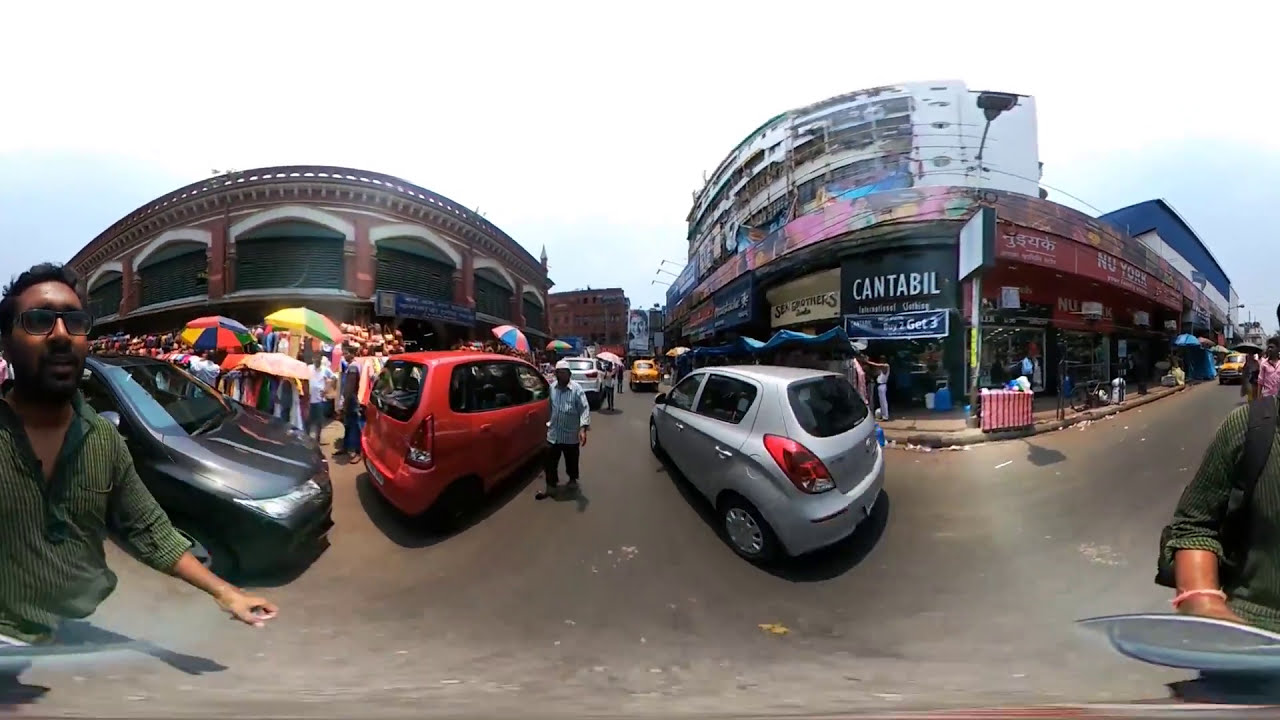The photograph captures a bustling street scene in a South Asian country, suggested by the various signs with foreign writing, including "N-U-Y-O-R-K" and "Canterbell." The view appears to be a panorama, evidenced by the slight distortion and the repetition of an Indian man with glasses and a button-down shirt walking towards the right, who is also partially visible on the far right side. The environment is urban but not modernized, featuring a mix of small, worn-down shops lined up next to each other with chipping paint and graffiti.

The left side of the image shows a crowd gathered under big, colorful umbrellas, possibly seeking shade from the sun, creating an impression of a communal or event-like atmosphere. Among the vehicles navigating through the alleyway, there is notably a taxi. The scene also includes a parking structure in the background, which is in a state of disrepair with battered rags and peeling facades.

The area suggests a low to middle-class setting. There are also some trash cans and signs promoting various items for sale. Notably, a camera is perched at the top, likely for monitoring the activities on the street. The varied elements—from the crowded hustle of people and vehicles to the vibrant signs and shop fronts—paint a vivid picture of everyday life in this South Asian urban locality.